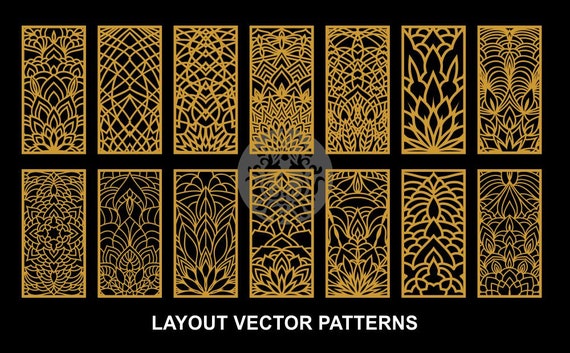The image showcases 14 examples of intricate layout vector patterns arranged in a 7x2 grid against a black background. Each pattern, depicted in gold line art, features geometric and mandala-like designs reminiscent of henna or lotus leaf motifs. The caption "Layout Vector Patterns" appears at the bottom in white text. A subtle circular logo, partially obscured and placed in the background, suggests the author's signature. The overall aesthetic bears a resemblance to Art Deco styles, characterized by angular and curved segments in the patterns.